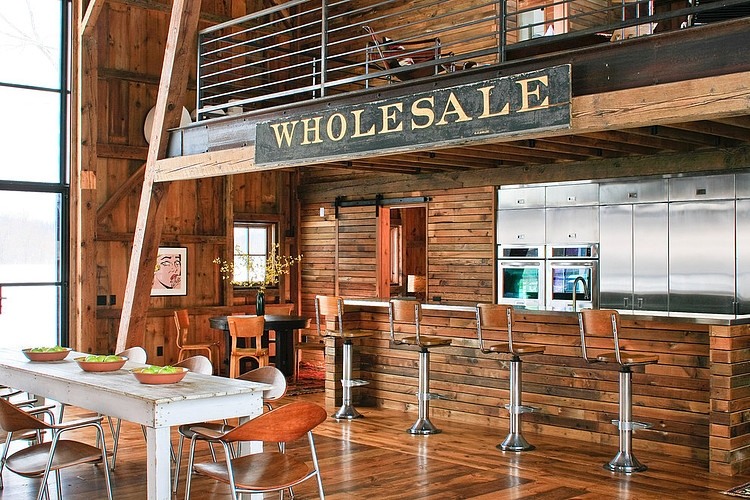The image is a detailed 3D color illustration of a cozy interior, likely depicting a kitchen, coffee shop, or restaurant setting. The scene features a two-level layout with a loft area above, characterized by dark wood floors and walls. The loft is secured with a black wrought iron railing. Just below this area, there's a prominent black sign displaying the word "wholesale" in white text.

On the bottom level, a modern and inviting ambiance is set with a sleek silver countertop accompanied by four bar stools that have wooden backs and seats, mounted on chrome pedestal posts. Adjacent to the counter, several stainless-steel kitchen appliances, potentially fridges or ovens, are neatly aligned against the wall. To the far left of this lower level, a long white wooden table is arranged with reddish-brown chairs, featuring concave seats and silver legs. The table is beautifully set with three round terracotta bowls filled with greenery.

In addition, there's a round black table with more brown chairs placed by a window, adorned with a black vase containing plants, enhancing the rustic yet modern decor. Completing the charming interior is a sliding barn door and a Roy Lichtenstein-style painting of a woman on one of the wood-paneled walls, adding an artistic touch to the space.